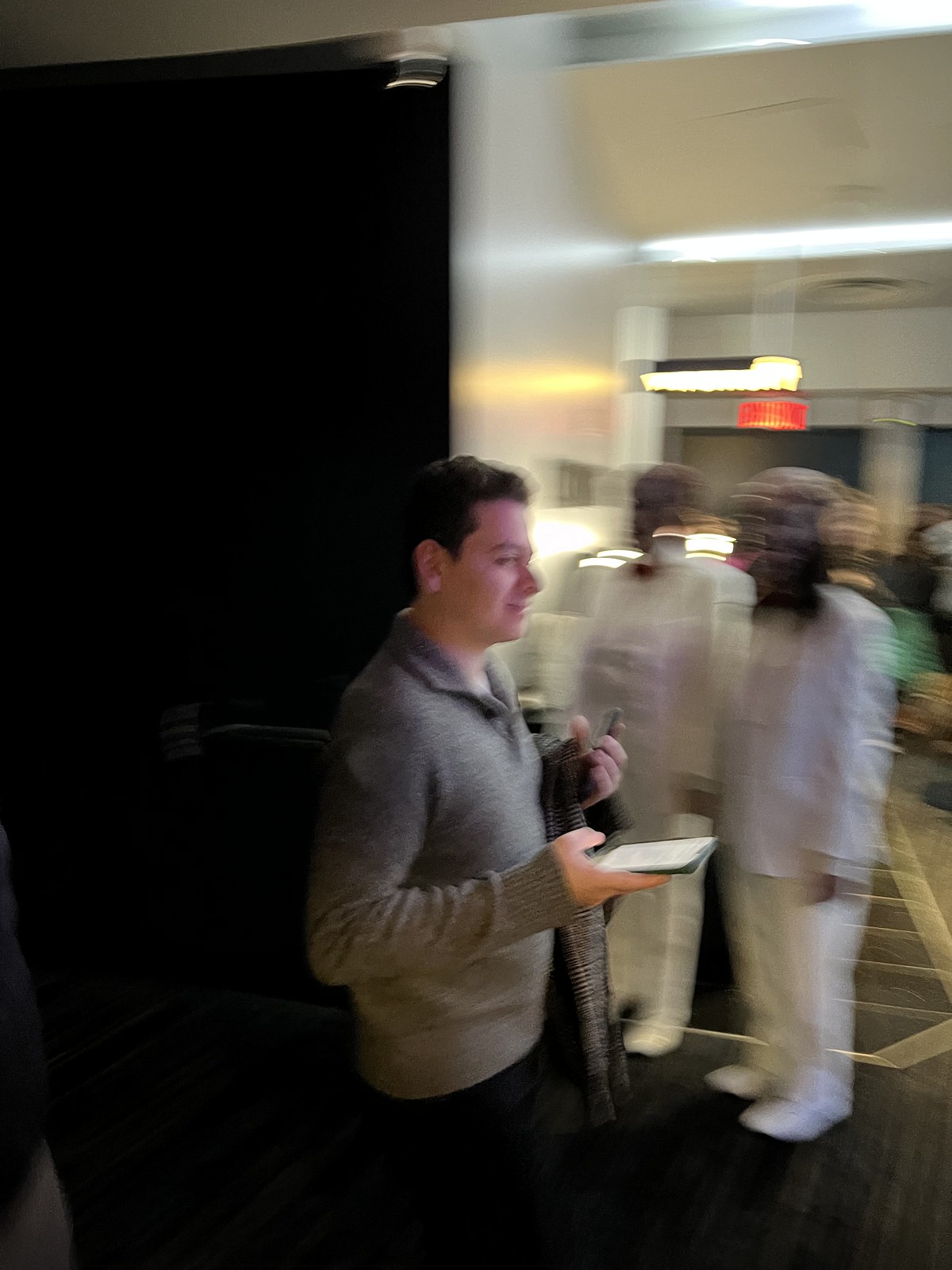A blurry image depicts two men, likely of Islamic faith, dressed entirely in white garments, complete with matching shoes, beards, and turbans. They stand outside, adjacent to a building that might be a place of worship. A passing white man, wearing a smug expression and glancing sideways at them, is holding an open phone as he walks by the scene, seemingly heading towards the building.